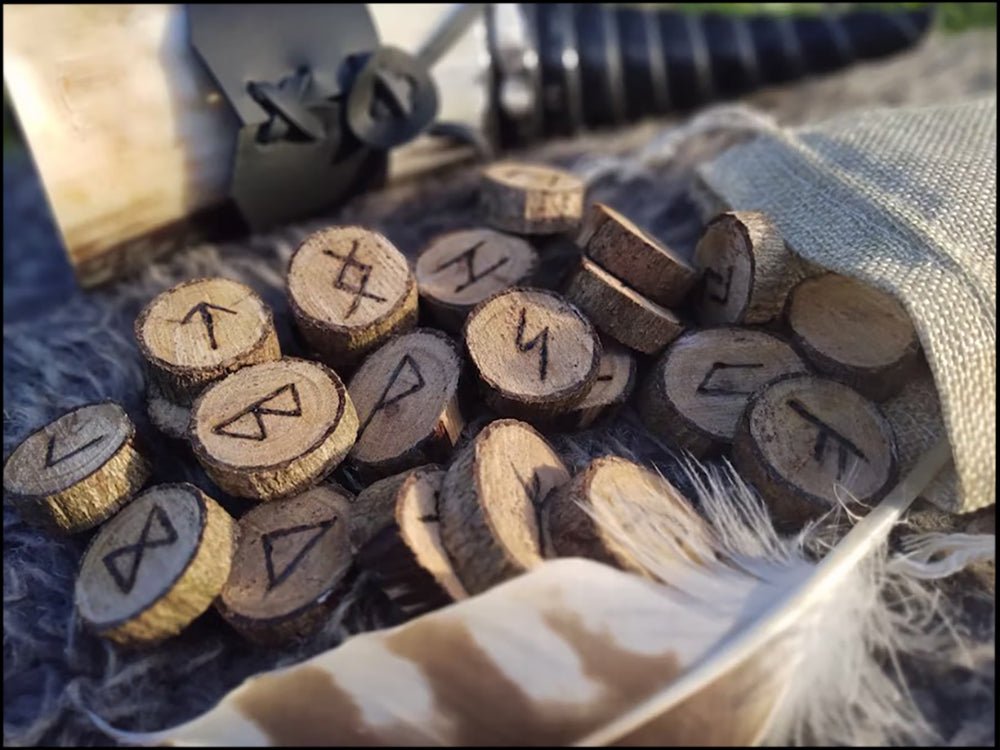The photograph captures an array of small wooden circles, which appear to be segments of a branch with bark still intact, each meticulously carved with Norse runes that resemble burnt markings. These wooden slices are scattered atop a fur-like surface, spilling out from a rough, tan burlap bag visible in the upper right corner. Additionally, a distinct feather, predominantly white with brown tints, possibly from a large bird, protrudes from the burlap bag, suggesting it might be used as a quill. Amidst this rustic setup, a black leather strap is discernible in the background, adding to the earthy, natural aesthetic of the composition. The arrangement evokes an image of ancient artifacts awaiting to be deciphered, all nestled in a scene reminiscent of a primitive, woodland setting.